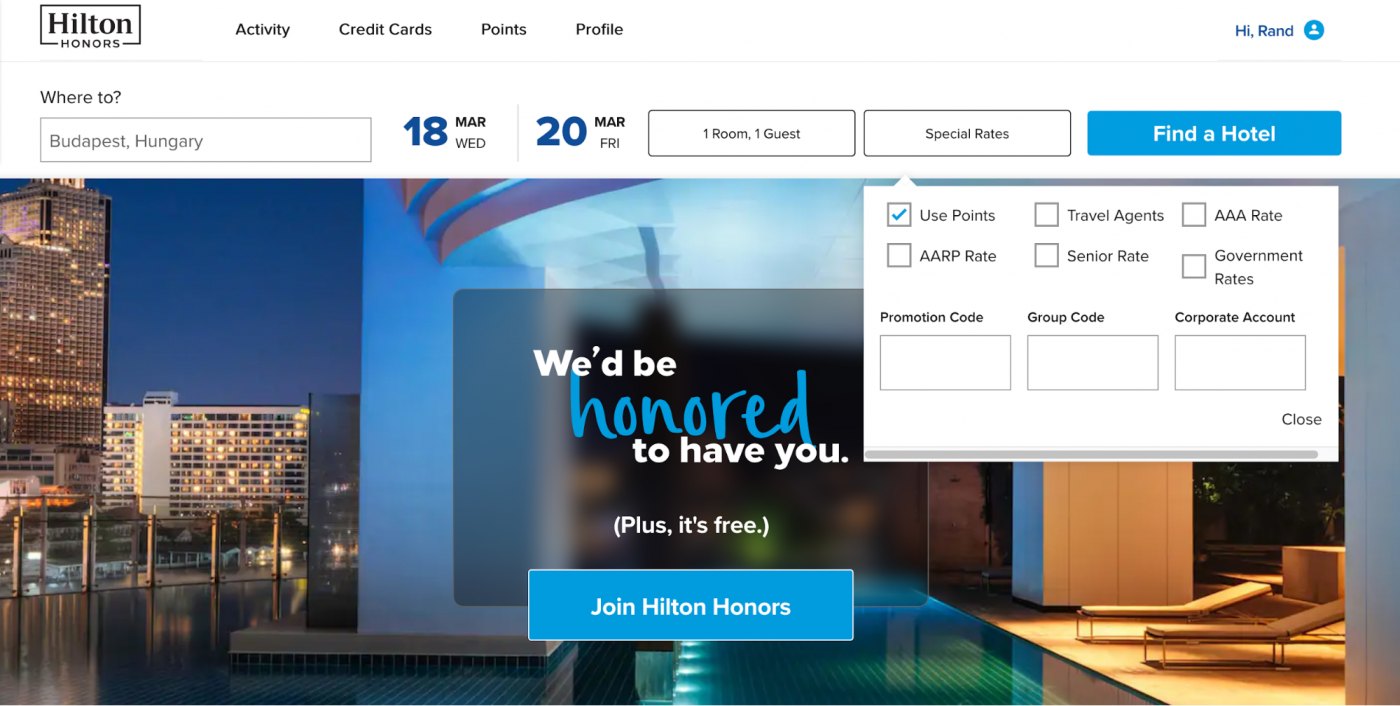The image showcases a webpage from the Hilton Honors loyalty program. In the top left corner, "Hilton Honors" is prominently displayed within a black box. On the right side, the website greets the user with "Hi Rand" in blue text, adjacent to a circular icon containing a silhouette of a person. Across the top, navigation options are available, including "Activity," "Credit Cards," "Points," and "Profile." 

Below the navigation bar, there's a search section starting with a prompt "Where to" followed by a field to enter a destination. Subsequently, there are fields to select the dates for check-in and check-out. Further down, options for rooms, special rates, and a blue "Find a Hotel" button are presented.

Under the "Special Rates" section, a dropdown box offers various rate options including "Use Points," "AARP Rate," "Travel Agents," "Senior Rate," "AAA Rate," and "Government Rates." Additional fields for entering promotion codes, group codes, and corporate accounts are also available.

Dominating the image is a scenic photograph featuring an inviting pool with lounge chairs in the foreground, set against a backdrop of a cityscape with several illuminated buildings. There's a vibrant blue sky visible in the distance. Overlaying this image is a message that reads, "We'd be honored to have you. Plus, it's free. Join Hilton Honors," encapsulated within a discrete call-to-action box.